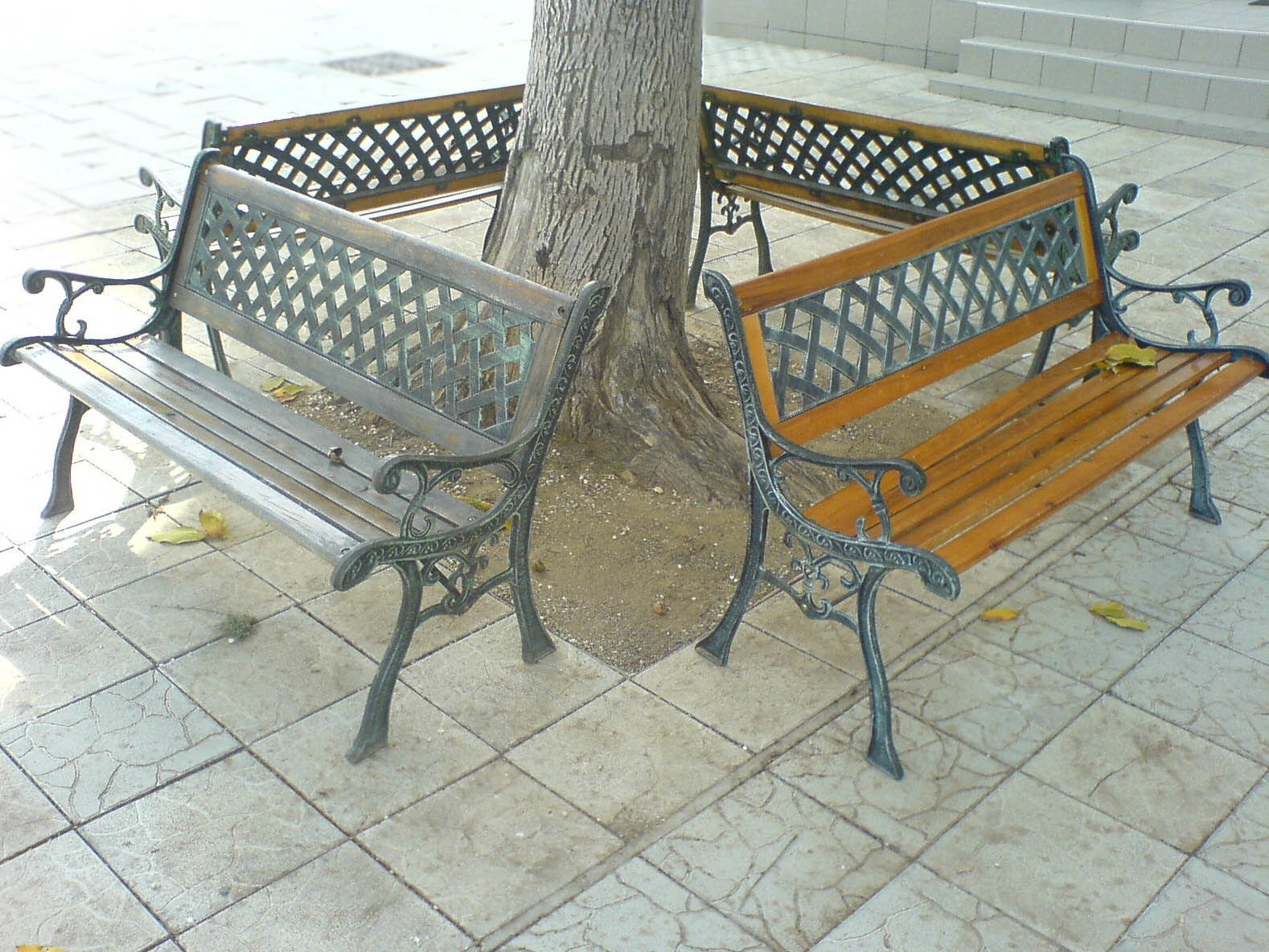The photograph captures a tranquil scene of a large tree growing out of a square plot of soil in a landscaped area, with its trunk surrounded by a grid of gray-brown pavers. Four wooden and metal park benches, arranged to form a square around the tree, are seen in the image. The benches have wooden seats and cast iron frames with a black paint finish, featuring intricate latticework designs on the backs and arms. The tree itself has its canopy cropped out of the frame, revealing only the solid, bare trunk. Notably, one bench appears weathered and worn, showcasing a duller, more jaded varnish in contrast to the others, which exhibit a newer, vibrant red-brown hue. In the background, three steps made of marble or stone are faintly visible, suggesting a slightly elevated area just outside of the main focus. The setting is devoid of people, emphasizing the stillness of the scene.